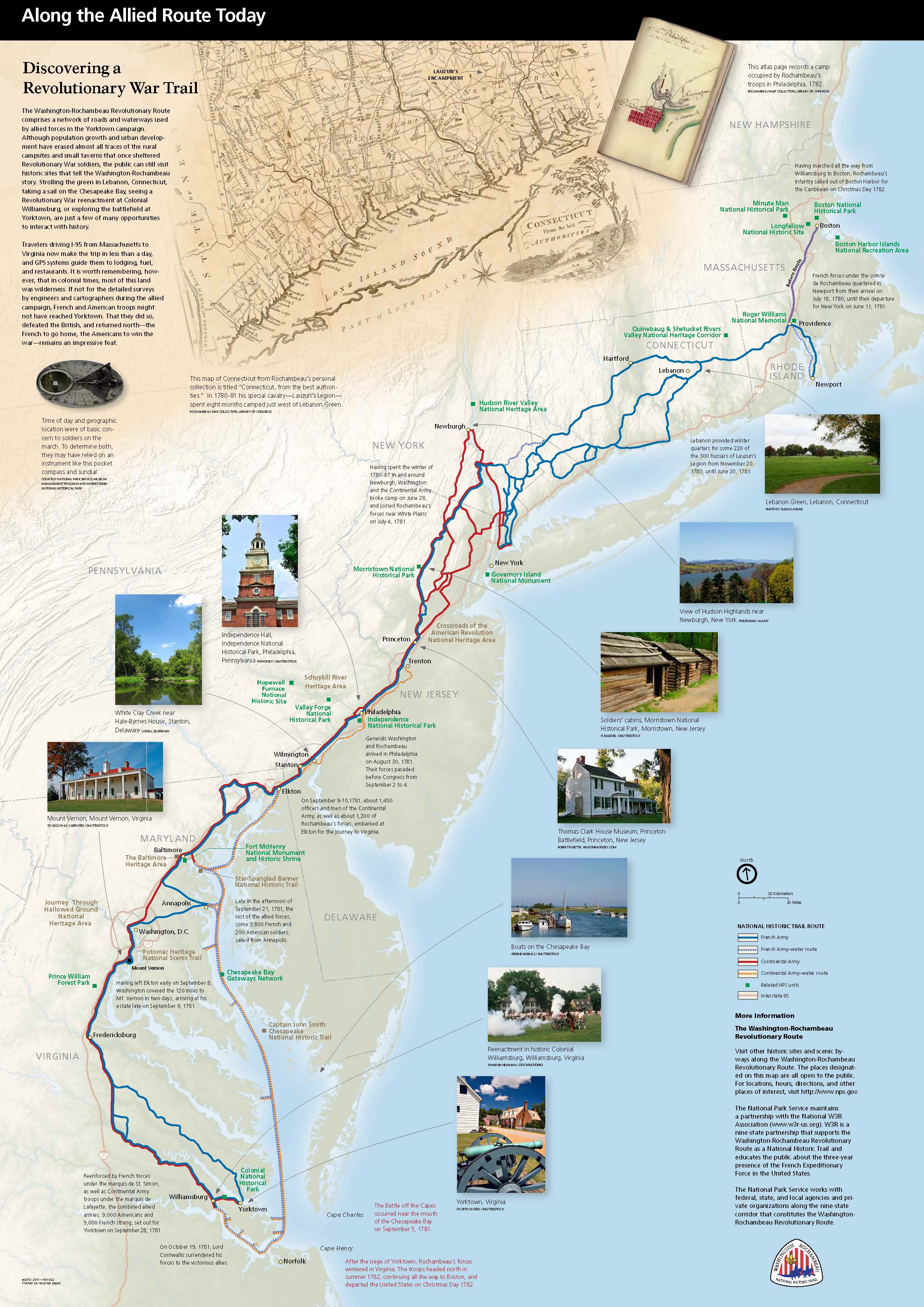The image resembles a highly detailed and informative page from a textbook or flyer, showcasing a comprehensive map of the east coast of the United States, specifically illustrating a Revolutionary War trail. At the top left, a black title with white text reads "Along the Allied Route Today," setting the historical context. Below this title, a heading, "Discovering a Revolutionary War Trail," precedes two paragraphs of explanatory text.

The map itself is tan-colored with topographical details and annotated with red and blue lines tracing the routes taken during the war, weaving near the land's edge and adjacent water bodies, predominantly to the right. Various landmarks and memorable events are denoted along these routes, each connected by arrows to corresponding colored photographs of key buildings and locations. These images and labels provide readers with visual and contextual references, making the trail's significance and path clearer. The overall layout is meticulously designed to occupy most of the page, emphasizing both the educational and visual aspects of the historic trail.